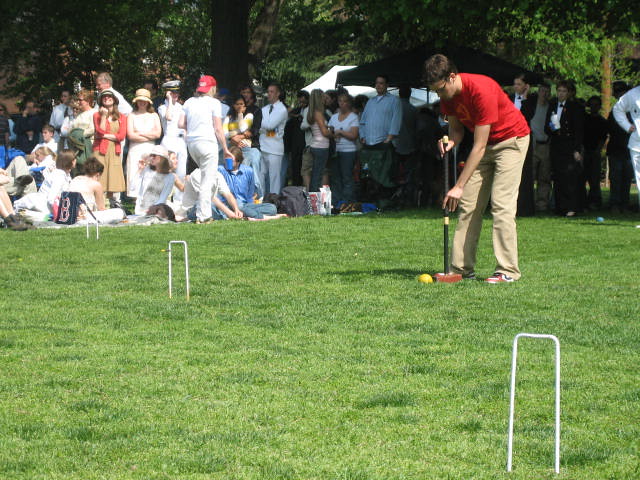The image captures a man intensely playing croquet, aiming to hit a yellow ball through the white metal wickets arranged on a lush green grassy field. He is wearing a red shirt, khaki pants, tennis shoes, and eyeglasses, with short brown hair. The man is positioned on the right side of the image, lining up his shot with a mallet featuring a red head and a dark handle with a stripe. 

In the background, about 10 feet away, a diverse group of spectators stands and sits in anticipation, suggesting this might be a tournament or championship event. Some individuals in the audience are dressed formally, with a few men donning black suits, black bow ties, and white dress shirts, and at least one man in a white suit. There are people standing underneath large trees providing shade, while others gather under a tent. Additional details include a man in a red ball cap, a woman in a uniform with an officer's hat, and two women wearing hats near the left-hand side of the image. The greenery and scattered trees add to the vibrant and lively atmosphere of the scene.